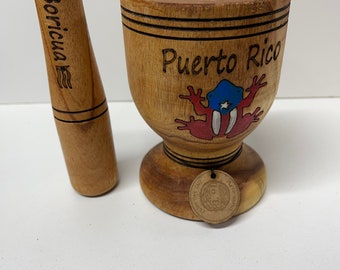This is a detailed image of a wooden mortar and pestle set, photographed against a white backdrop and placed on a white table, giving it a studio-like environment. The set appears to be crafted from brown wood with intricate details. The mortar, prominently displayed, features three black engraved lines near its rim with the word "Puerto Rico" inscribed below. Accompanying the text, there is an illustrative frog adorned with the Puerto Rican flag, which is red with white stripes, a blue head, and a white star. At the base of the mortar, a white string is wrapped around, holding a wooden medallion with an indistinct pattern. To the left, the pestle follows the same wooden aesthetic, bearing two engraved black lines and the word "Boricua" along its length. Although the top parts of both items are not visible, the visual details and inscriptions provide a rich cultural context, emphasizing their Puerto Rican heritage.